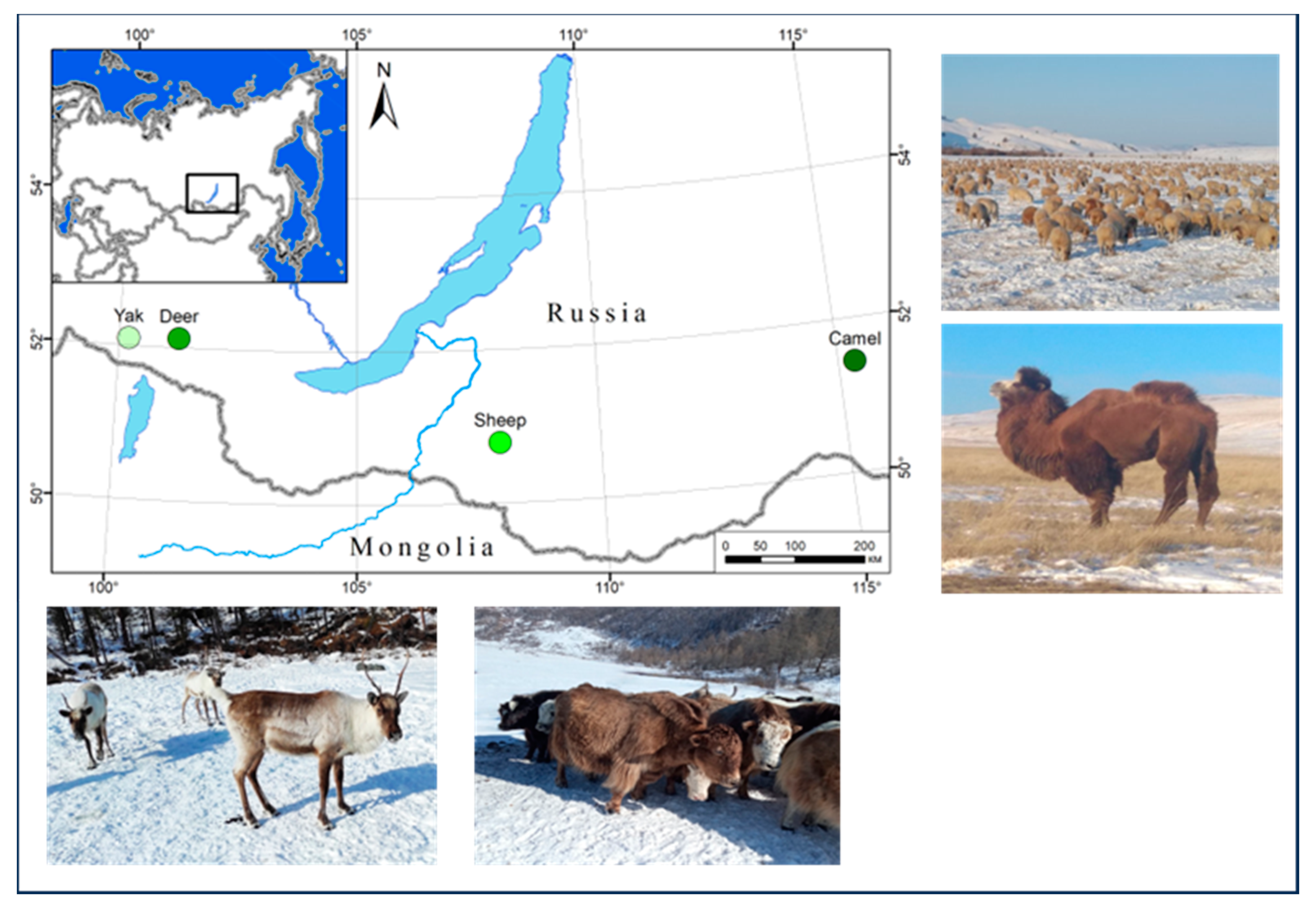The image is a detailed geographic illustration highlighting the locations and habitats of certain animals along the Russia-Mongolia border. 

In the top left corner is a primary map of this border area, supplemented by an inset map for broader continental context. The border is denoted by a gray line, and specific locations within Russia are marked with different shaded green dots indicating where a yak, deer, sheep, and camel were found. The map also features longitude lines marked with degree symbols, such as 100°, 105°, 110°, and 115°.

Surrounding this map, there are four photographs of the animals in their natural habitats. In the top right is an image of brown-furred sheep in a snowy flat plain with some distant hills. Below this, there is a picture of a brown camel standing in a sunny tundra area where the snow appears to be melting. On the bottom left, there is a group of white and brown deer set against a snowy background with some visible trees. To the right of this, there are images of yaks in a similarly snowy environment.

Overall, this visually informative diagram offers a snapshot of where these animals are located in Russia, showing detailed imagery for better understanding and identification.